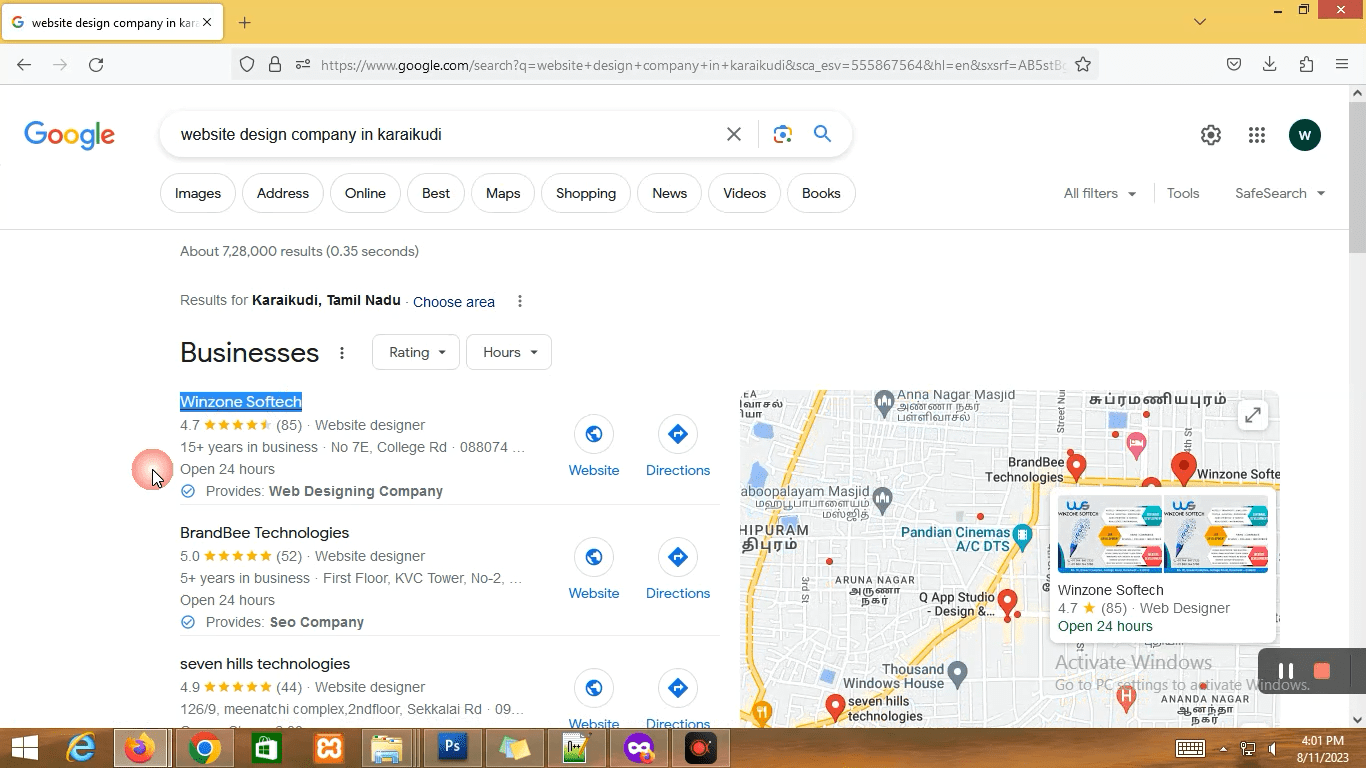This image captures a screenshot of a Google search results page for the query "Website Design Company in Karaikudi." The results page is well-organized, with approximately 7,028,000 results displayed in just 0.35 seconds. Positioned directly beneath the search bar are eight filter tags: Images, Address, Online, Best, Maps, Shopping, News, Videos, and Books.

The search results prominently feature three businesses specializing in website design:

1. **WinZone SoftTech**
   - Rating: 4.7 stars
   - Reviews: 85 ratings
   - Experience: Over 15 years
   - Availability: Open 24 hours
   - Links: Website and Directions

2. **BrandB Technologies**
   - Rating: 5 stars
   - Reviews: 52 ratings
   - Experience: Over 5 years
   - Availability: Open 24 hours
   - Specialty: CEO company
   - Links: Website and Directions

3. **Seven Hills Technologies**
   - Rating: 4.9 stars
   - Reviews: 44 ratings
   - Links: Website and Directions

Located on the right side of the page is a map showing the geographic details of Karaikudi in Tamil Nadu. The map prominently features a pop-up window highlighting WinZone SoftTech’s location. A rating system and operational hours are indicated for each business, and all listings include both website links and directions to their respective offices.